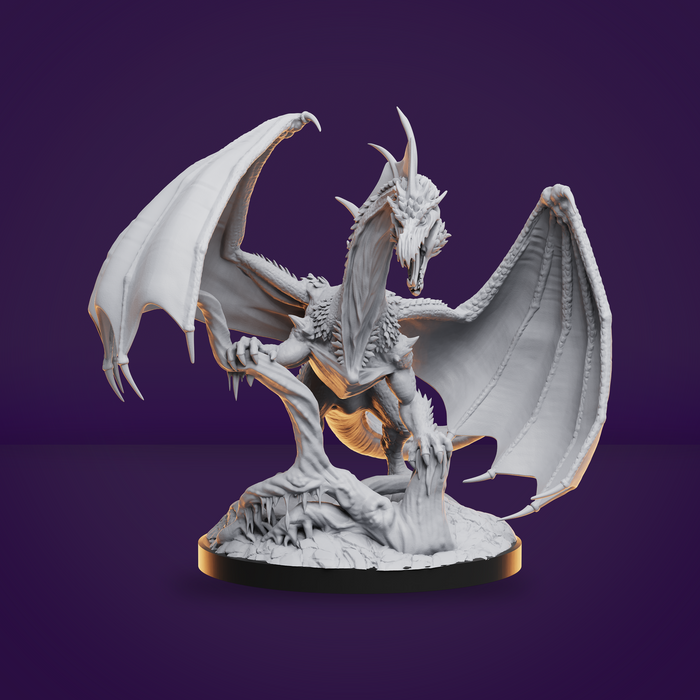This detailed sculpture of a menacing white dragon, likely 3D-printed, features highly intricate and fine details. The dragon, with large bat-like wings spread wide, shows a pattern typical of 3D printing. The wings have spike-like points resembling teeth. The fierce dragon appears to be roaring, revealing sharp teeth and a complex array of scales and horns from its chest upwards. It stands powerfully on a white, melting tree trunk with its muscular arms, adorned with large claws gripping the tree. The base of the sculpture is a striking gold-copper color, adding a rich contrast. The display is set against a purple background and table, suggesting a studio setup, with the entire image maintaining a square frame. Gold highlights and an orange underglow enhance the sculpture, adding depth and visual interest to the scene.